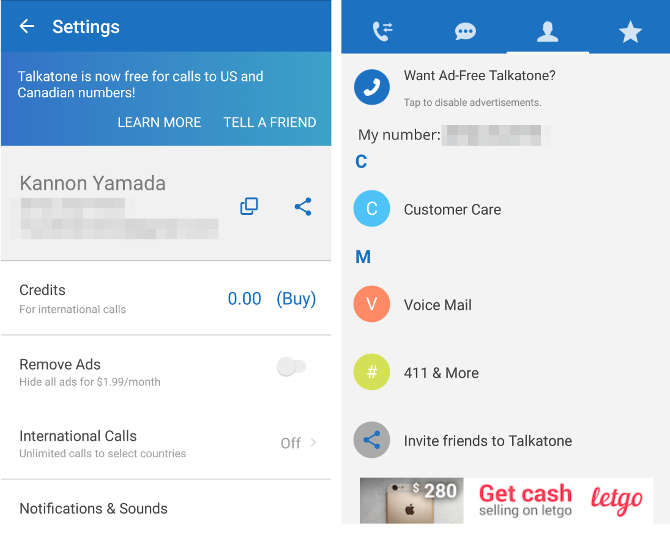This pair of screenshots showcases different sections of a mobile app's settings and main interface.

In the first screenshot titled "Settings," a back arrow is visible at the top left corner. The main content announces that TalkTone now offers free calls to US and Canadian numbers. Below this announcement, users can choose to either "Learn More" or "Tell a Friend." The section under "Canon Yamda" highlights the user's current credits for international calls, showing a balance of zero with an option to "Buy" more credits. Additionally, there is an option labeled "Remove Ads," priced at $1.99 per month, which is currently turned off. Another inactive toggle is present for "Unlimited Calls to Select Countries." This page also has options for configuring "Notifications and Sounds."

The second screenshot captures the main interface of the app, characterized by a blue banner at the top. This interface features multiple tabs along the bottom, including icons for calling, messaging, contacts, and favorites. A line beneath the "Contacts" tab indicates it is the active page. Displayed within this tab are various contacts such as "Customer Care," "Voicemail," and "411," although the user's personal number appearing is blurred for privacy. An advertisement for LetGo, a selling platform, appears at the bottom, featuring a red LetGo icon with the message "Get cash selling on LetGo."

These screenshots collectively illustrate the app's functionalities with details on available services, settings customization, and user interface layout.